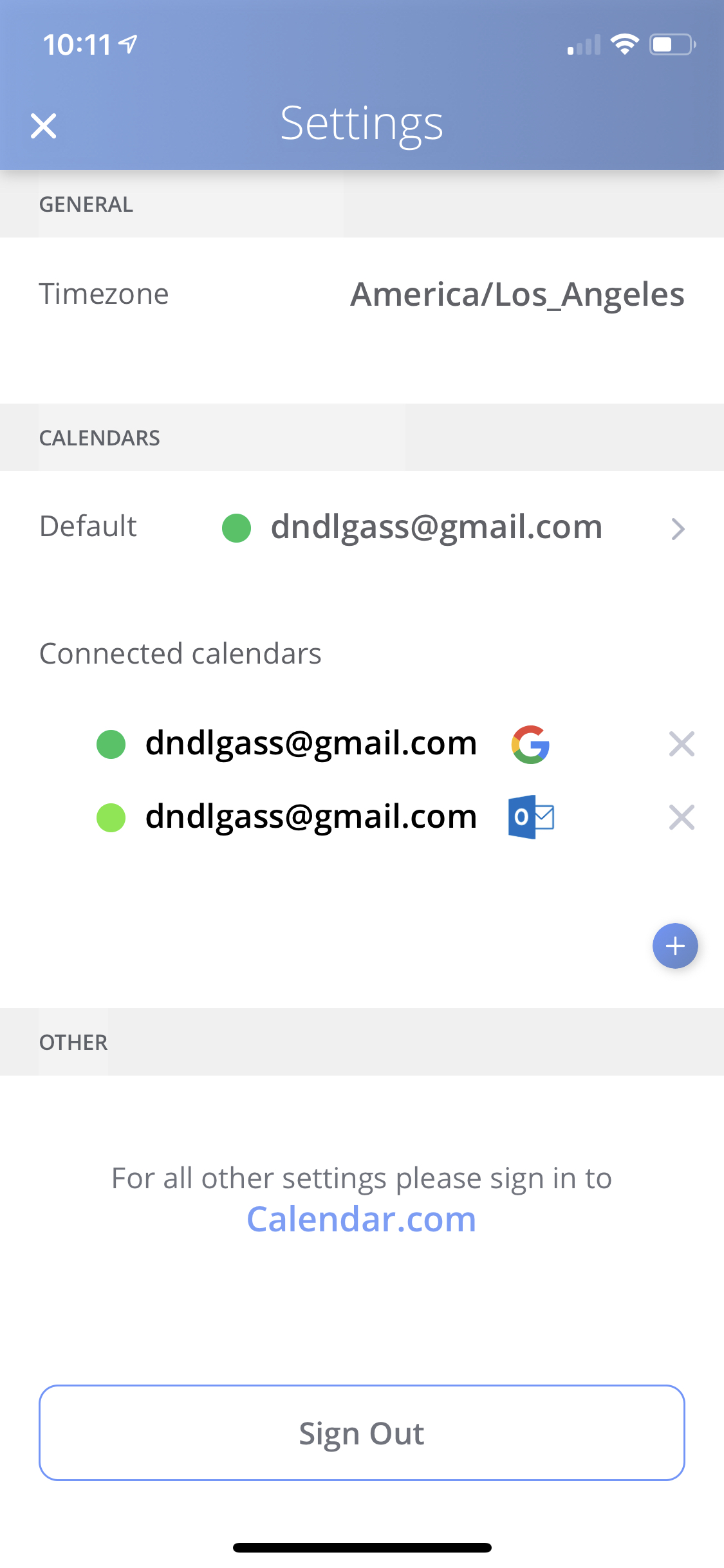The image displays a digital interface highlighting various settings and options. 

In the top left corner, the time is shown as 10:11. To the right of the time, there is a battery icon indicating a half charge. Central to the header, the word "Settings" is prominently displayed. On the far right, an "X" icon is visible, likely for closing the settings menu.

Directly beneath this header is the word "GENERAL" in uppercase letters, followed by the option "Time Zone." To the right of "Time Zone," the text "America/Los_Angeles" indicates the selected time zone.

The next section is labeled "Calendars." Below this heading, the word "Default" is shown with a green circle to the right, followed by the email address "DNDLGASS@gmail.com." Moving further down, it reads "Connected Calendars," and again, a green circle is present next to the identical email address "DNDLGASS@gmail.com."

Below this, the same email address "DNDLGASS@gmail.com" appears once more, this time accompanied by a blue square with an envelope icon to the right. Additionally, a blue circle with a plus sign is shown, likely for adding another item. Next to it, a long rectangle contains the word "Other."

At the bottom of the section, there is an instruction in blue text: "For all other settings, please sign in to calendar.com." 

Approximately three inches further down is a blue-outlined rectangle with the words "Sign Out" inside.